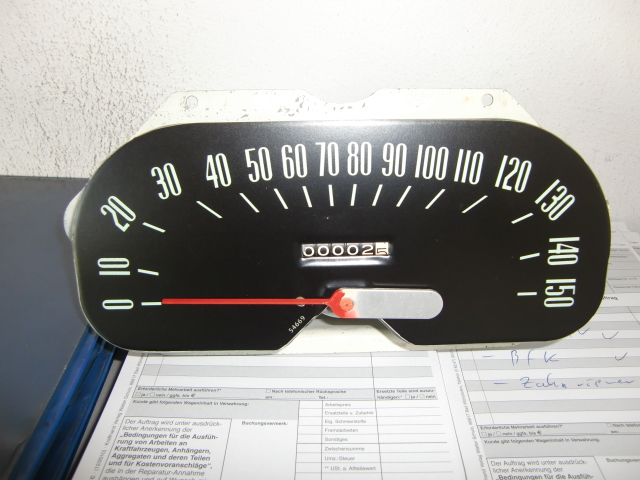This vibrant color photograph features a black analog scale with a detailed numeric display and various markings. The scale's numbers, ranging from 0 to 150 in increments of 10, are written in white with corresponding dashes beneath each one. As the focal point of the image, a long red pointer, which adjusts according to the weight measured, is positioned in the foreground. Above the scale's numbers, an odometer-style wheel displays the digits "0, 0, 0, 0, 2, 0.5."

Beneath the scale, there is paperwork that resembles a medical chart, complete with various boxes designed for input. This paperwork, featuring text in a different language, has black writing and checkmarks on the right-hand side. The document's gray and white hues contrast subtly with its black lettering. Everything rests on a gray table, and the backdrop includes a lighter gray, textured wall, providing a neutral background that highlights the scale and accompanying documentation.